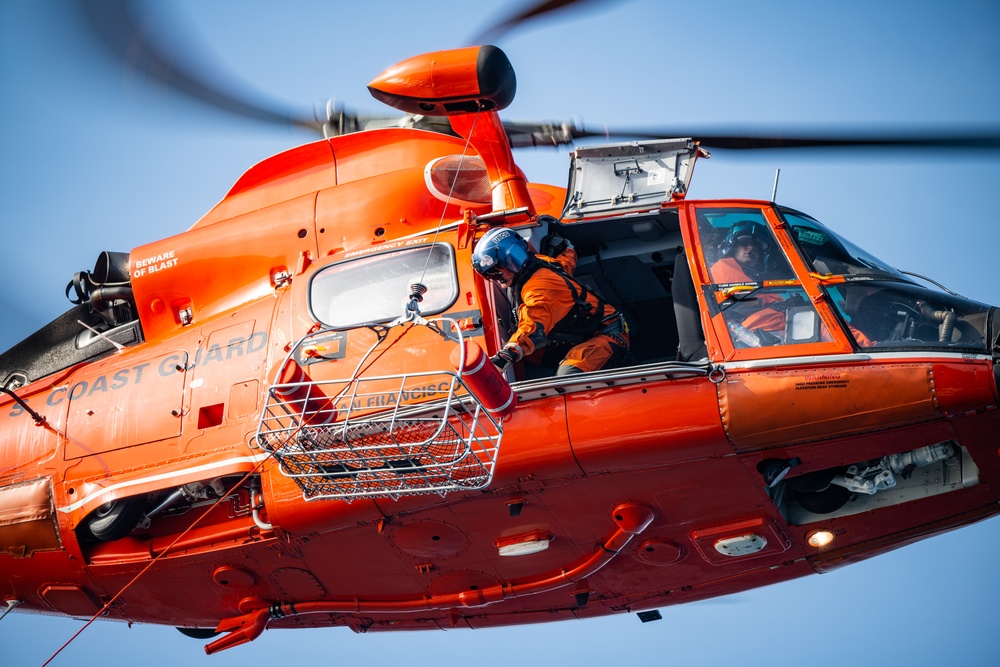This image captures a dramatic mid-air scene during the daytime, featuring a deep orange Coast Guard helicopter orchestrating a rescue operation high in the sky against a backdrop of a clear, light blue horizon. The helicopter's propeller blades, spinning at high speed, create blurred, curved black lines over the top left and straight across the top right of the frame. This rectangular photograph, approximately six inches wide by four inches high, provides an angled view from slightly below, possibly taken by a drone or another aircraft.

The nose of the helicopter extends to the right-hand side of the image, although it remains just out of frame. The aircraft's landing gear is retracted. Both the pilot, visible through a slightly tinted window, and a second Coast Guard worker, who is leaning out of the open side door in an orange jumpsuit and silver helmet, are intently focused on the operation. This worker is maneuvering a white rescue basket attached to a cord, positioned to be lowered, likely as part of a rescue effort. The basket appears to have flotation devices on either end, typical of equipment used in sea rescues.

Prominently displayed on the rear left side of the helicopter's fuselage are the words "Coast Guard" in dark gray print. The tail of the helicopter extends out of the frame on the left side. The sense of urgency and purpose is palpable, accentuated by the detailed realism captured in the photograph.